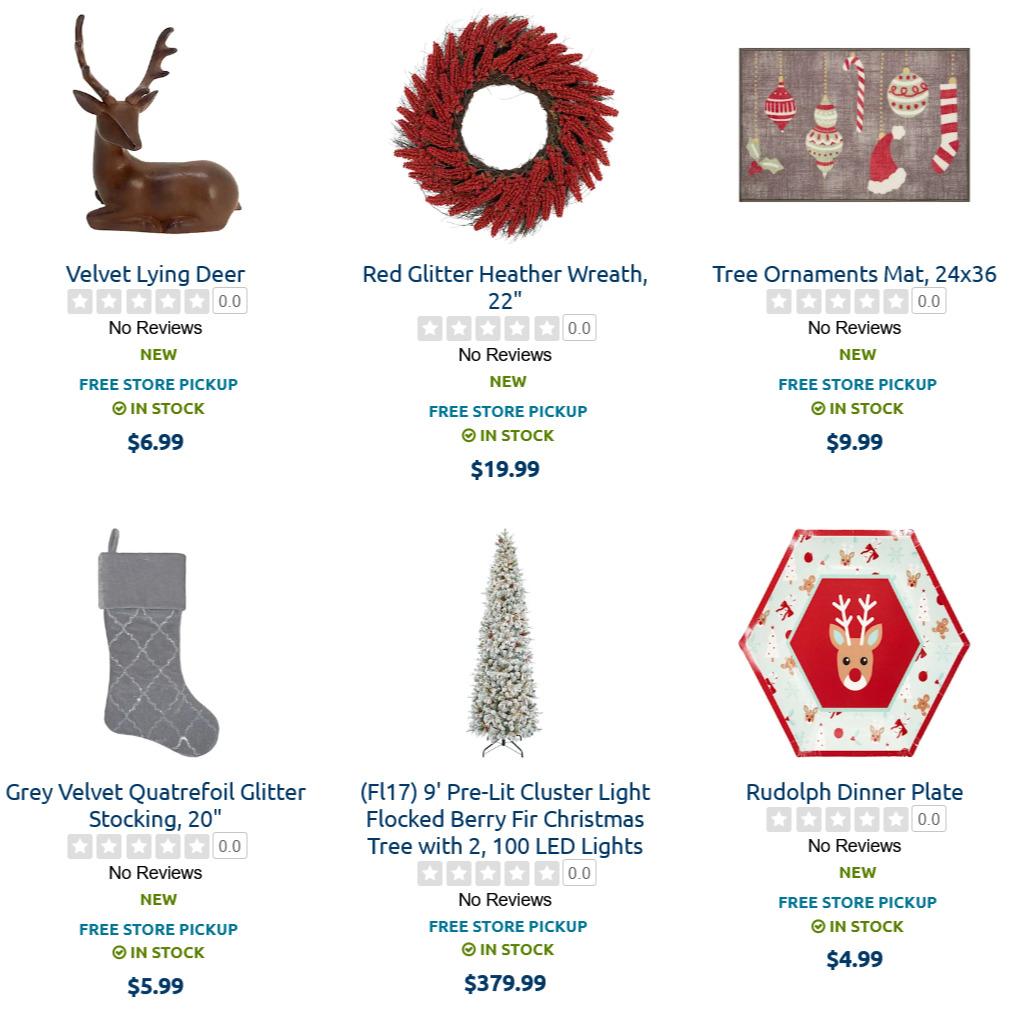This image depicts a store page from an unidentified website featuring an array of Christmas items. From left to right and top to bottom, the items include:

1. A Velvet Laying Reindeer Figurine: This brown reindeer decoration is made of velvet and is priced at $6.99. It is available for free store pickup and currently has no reviews or star ratings.

2. A Red Glitter Heather Wreath: A 22-inch red wreath adorned with glitter. This new item is also available for free store pickup, priced at $19.99. It currently has no reviews or star ratings.

3. A Christmas Ornaments Welcome Mat: Measuring 24 by 36 inches, this gray welcome mat features a design with Christmas ornaments. It is priced at $9.99 and has no reviews or star ratings.

4. A Gray Velvet Glitter Stocking: This 20-inch stocking is gray with glitter accents and is priced at $5.99. It is currently available for free store pickup and has no reviews or star ratings.

5. A 9-Foot Pre-Lit Cluster Light Flocked Berry Garland: This extensive garland is designed for Christmas trees and includes 2,100 LED lights. The item is priced at $379.99 and has no reviews or star ratings.

6. A Rudolph Dinner Plate: This festive red plate features an image of Rudolph the Red-Nosed Reindeer in the center. It is priced at $4.99 and has no reviews or star ratings.

Each item on this page is in stock and available for free store pickup, albeit with no customer reviews or ratings.